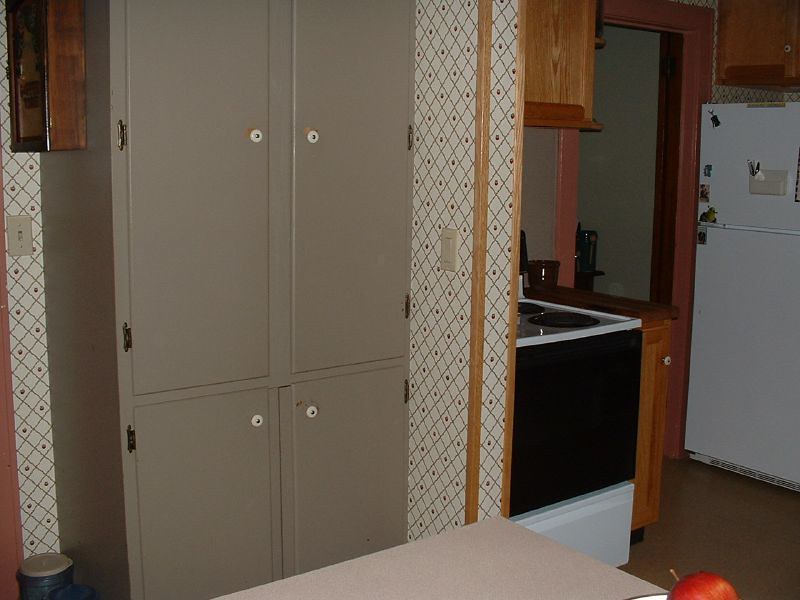This image depicts an old-fashioned, indoor kitchen. Upon entering from the left, the walls are adorned with white wallpaper featuring black diamond shapes, some containing black dots. Adjacent to this wall stands a tall, gray cabinet with four doors, accented by white handles with silver inserts and visible gold hinges. Directly in front of this cabinet is a countertop or kitchen island with a light pink to tan surface, upon which sits a white bowl containing a single red apple with a brown stem.

To the right of this setup, the kitchen layout continues with wooden cabinetry above and below counter level, providing ample storage space. The wooden cabinets match the wood grain seen throughout the room, including the door frames and possible trim. On the far right of the image, a white refrigerator is adorned with a few magnets, including a green "Shrek" character, and a small holder containing pens.

The kitchen also features an older-style electric stove with a white stovetop and black oven door. The stovetop has black coil burners, typical of older electric ranges. Above the stove, there is another wooden cabinet or possibly a fan hood.

The room spills into another section, suggesting an open floor plan. Through the open doorway to the left of the refrigerator, a room is visible with a darker ambiance and possibly a green backdrop. Additionally, there's a visible light switch and a border of wood trim that adds to the old-fashioned charm of the kitchen. The overall color palette includes various shades of brown from the cabinetry, white from the refrigerator and stove, and a touch of red from the apple, creating a warm and somewhat dated aesthetic.